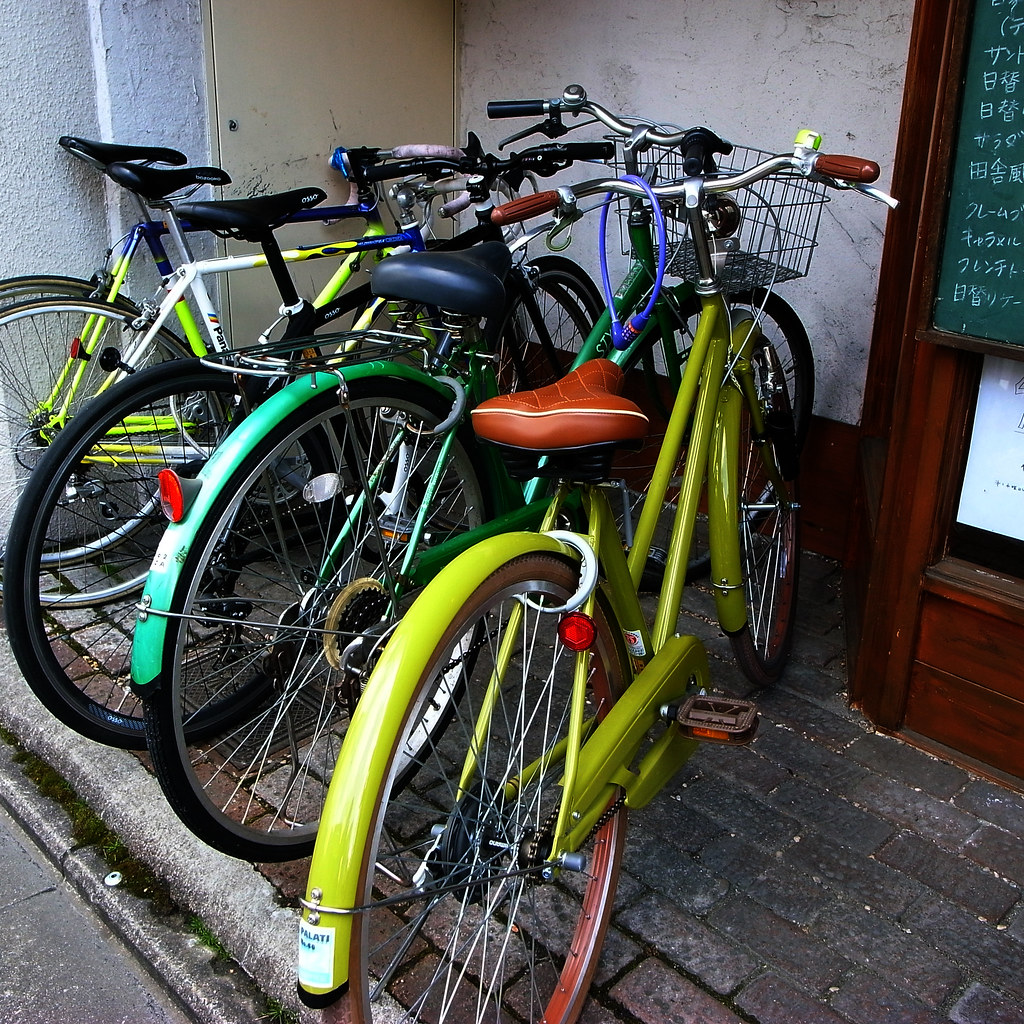This photograph, captured outdoors on a somewhat cloudy day, depicts five vibrantly colored bicycles parked in front of a storefront on a dark cobblestone sidewalk. The storefront has a tan wall with a dark brown wooden door, which features a chalkboard sign with Chinese characters, possibly indicating a menu for a restaurant or shop. The first bicycle on the right is a striking lime green with a tan leather seat and big brown-trimmed handlebars. The next one is a kelly green bike with a black seat and a green fender. There's also an all-black bicycle, a yellow and blue racing bike with a high black seat, and another yellowish green bike with a brown-orange seat. One of the bicycles features a wire wicker basket on the front, while another has a racket hanging off its handle. The bicycles appear to be loosely locked together with bike locks visible around some of the handlebars, and they are aligned with their front wheels facing the building. The bright colors of the bikes stand out against the cobblestone pavement and the brick sidewalk, adding a vibrant splash to the scene.